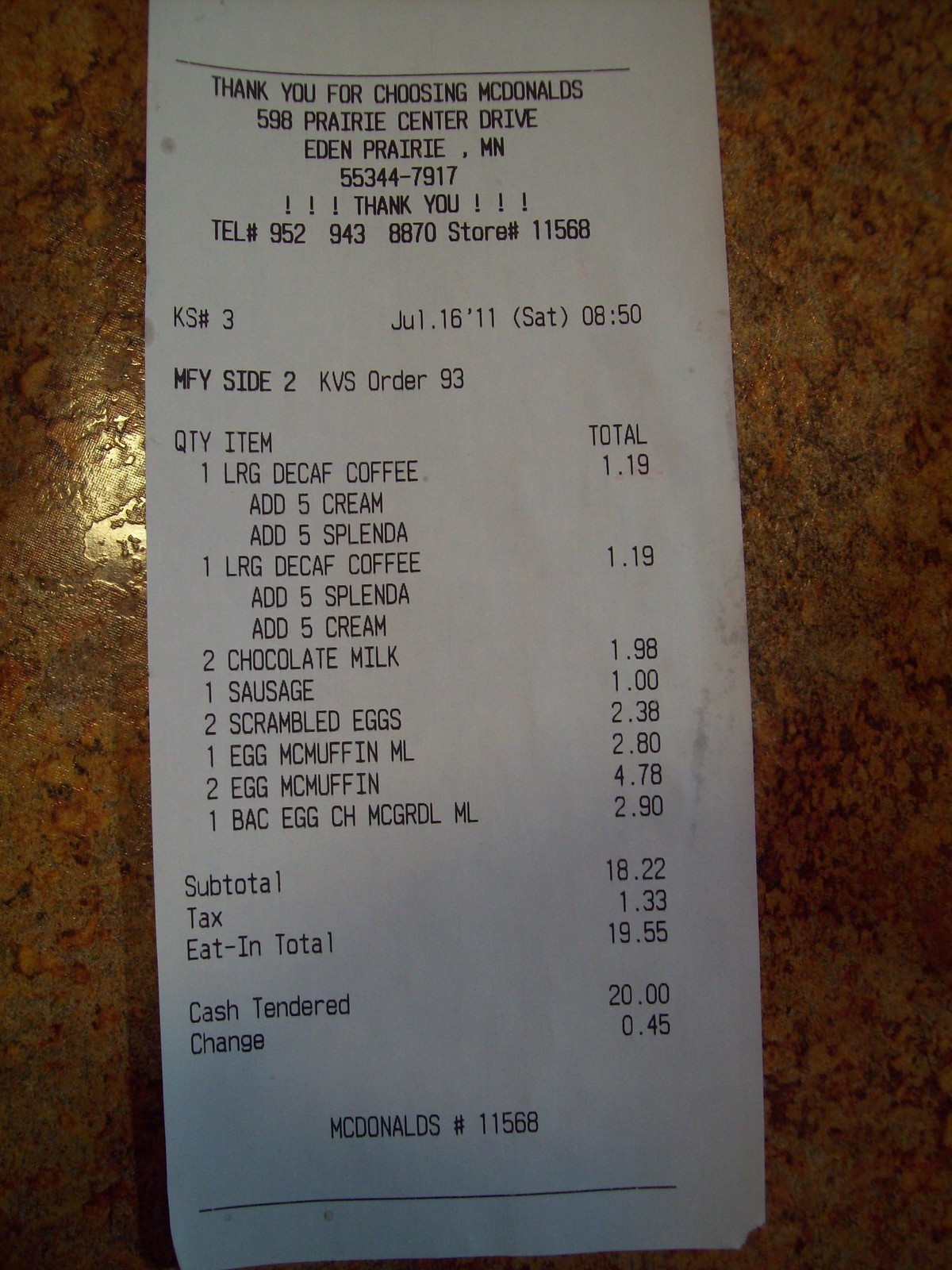This is a close-up photograph of a long, white grocery receipt with black text, placed on a dark brown table that features black, light brown, and beige specks. The receipt is from McDonald's located at 598 Prairie Center Drive, Eden Prairie, Minnesota, 55344-7917. It was issued on July 16, 2011, at 8:50 AM. The store number is 11568, and the telephone number is 952-943-8870.

The receipt details the following purchases:

- One large decaf coffee with five creams and five Splenda for $1.19
- Another large coffee with five creams and five Splenda for $1.19
- Two chocolate milks for $1.98
- One sausage for $1.00
- Two scrambled eggs for $2.38
- One Egg McMuffin for $2.80
- Two Egg McMuffins for $4.78
- One Bacon Egg and Cheese McGriddle for $2.90

The subtotal for these items is $18.22, with a tax of $1.33, bringing the total to $19.55. The payment was made with a $20 bill, resulting in a change of $0.45. The receipt expresses gratitude with "Thank you for choosing McDonald's" included at the top and bottom, along with three exclamation marks on either side.